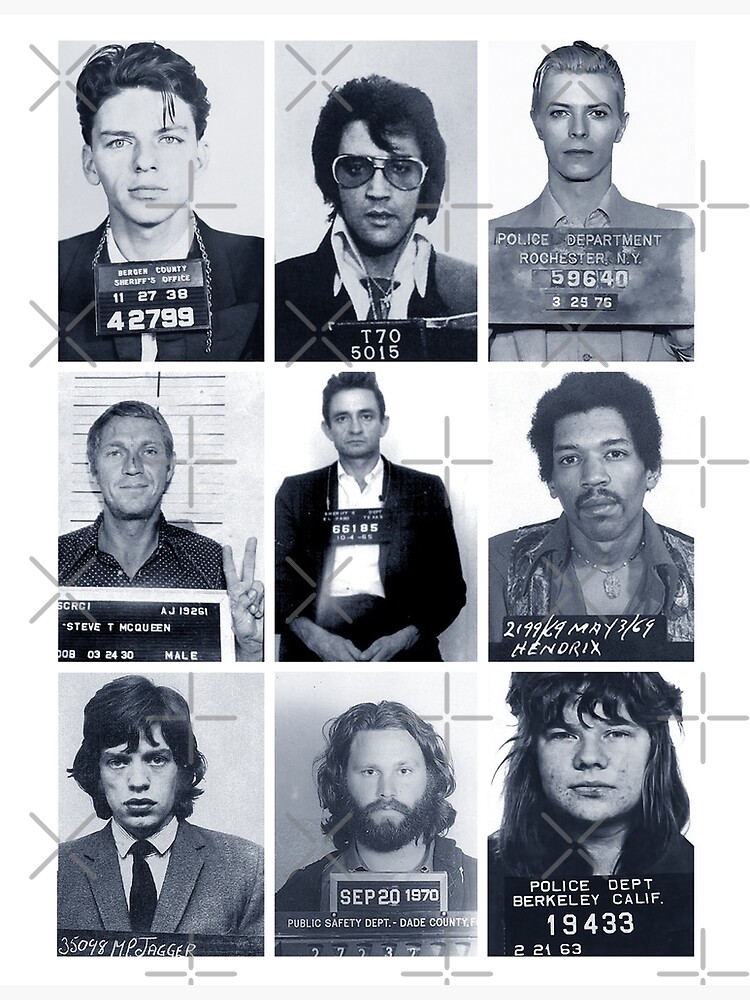The black-and-white image features a three-by-three grid of famous celebrity mugshots, each marked with watermarks of plus and X symbols. In the top row, from left to right, are Frank Sinatra, Elvis Presley, and David Bowie. The middle row showcases Steve McQueen, Johnny Cash, and Jimi Hendrix. The bottom row includes Mick Jagger, Jim Morrison, and, in the bottom right corner, what appears to be Janis Joplin, with a mugshot dated from Berkeley, California, 1963. Each mugshot is a poignant reminder of the storied and sometimes tumultuous lives of these iconic figures.